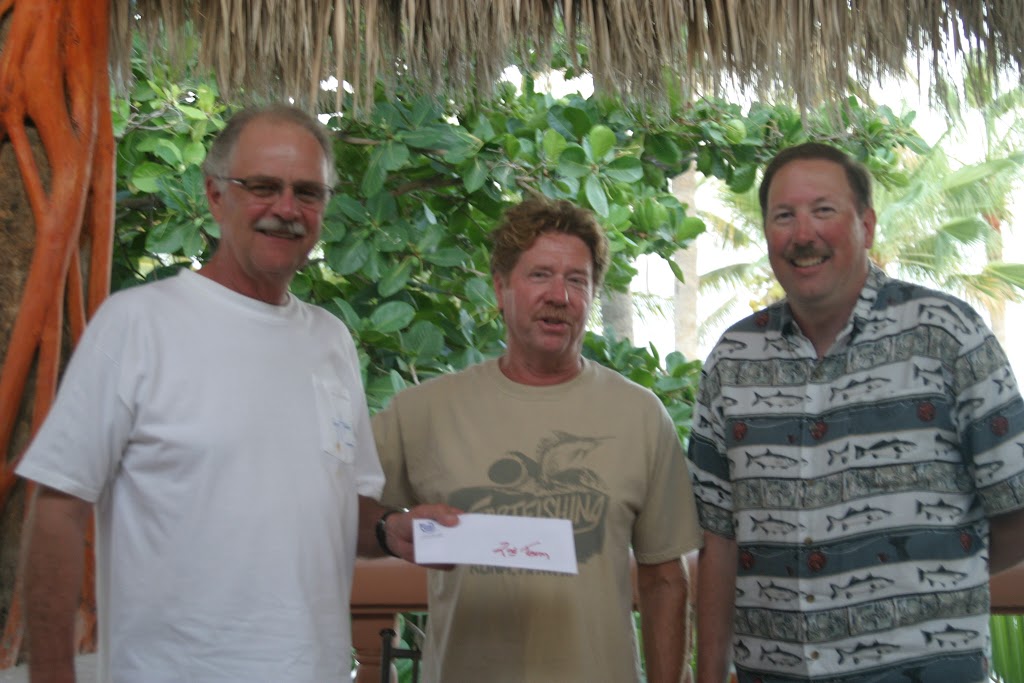In the photograph, three middle-aged men, all wearing casual shirts, stand together under a gazebo adorned with dried palm leaves, surrounded by lush, leafy vegetation and a distant wooden fence that suggests a warm, possibly tropical climate. Each man is smiling broadly, appearing very happy. The man on the left wears a white t-shirt with a pocket, adorned with blue lettering, and holds a white envelope with red lettering in his left hand. The man in the middle, clad in a beige t-shirt featuring an advertisement and a depiction of what looks like a swordfish, has sandy blonde curly hair. The man on the right sports a colorful short-sleeved shirt with fish-patterned gray stripes, along with a mustache and receding dark brown hair. The central figure is visibly holding what seems to be a check, though the details of the check remain unreadable. The scene captures the joyful moment of the presentation, likely commemorating a donation or special cause.